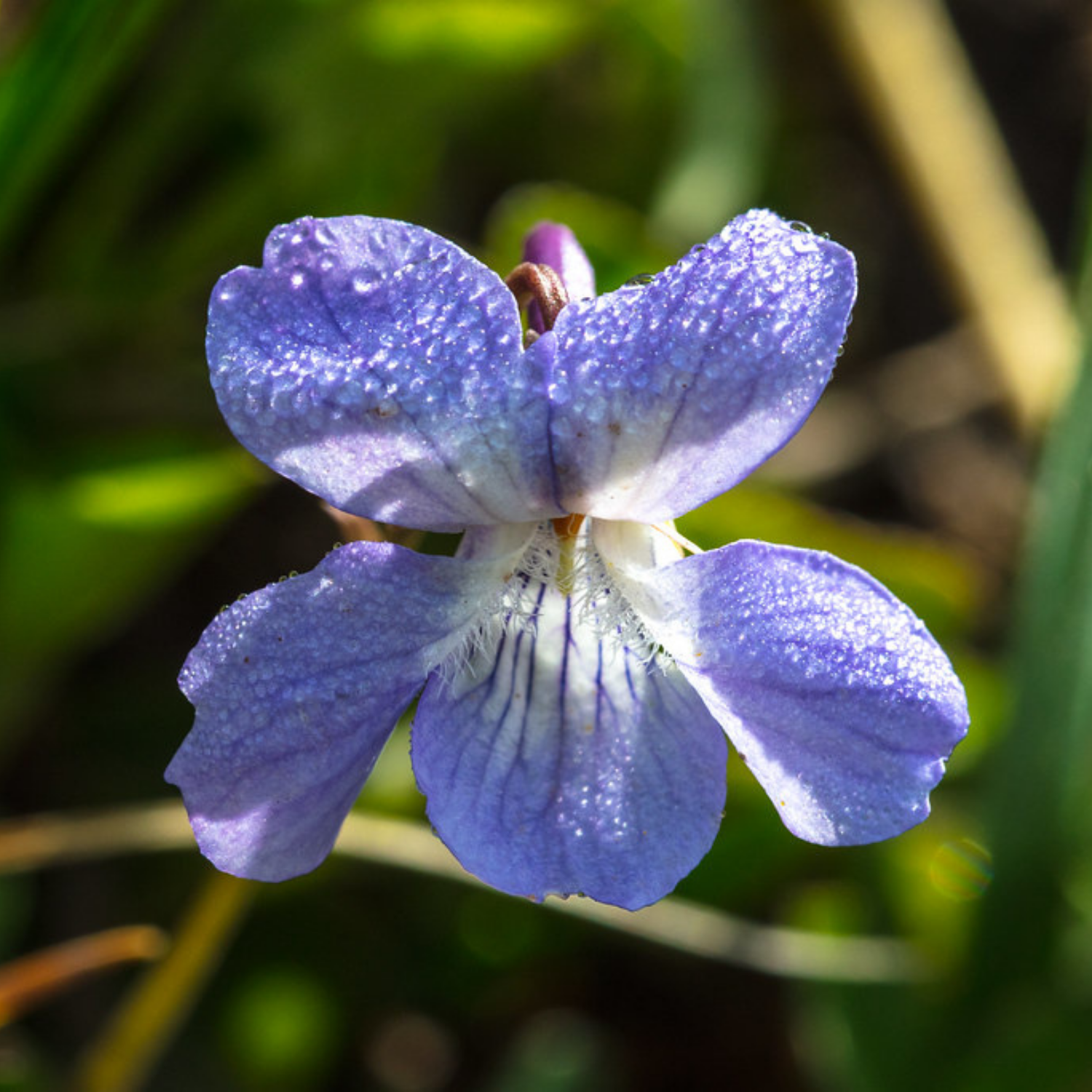This detailed close-up image captures a stunning blue flower, most likely a wild violet or possibly an orchid, with five petals and a vibrant yellow center. The delicate petals, displaying intricate darker blue veins that radiate towards the center, are adorned with glistening dew drops, emphasizing the freshness of the early morning or a recent rain. The flower has a unique arrangement: two petals on top and three on the bottom, with the central bottom petal being the largest. The background is a soft blur of dark green and occasional purple, suggesting other vegetation and possibly additional flowers, which accentuates the main flower's vivid details and colors, including hints of light blue, violet, yellow, purple, green, and a touch of brown. Set against this out-of-focus backdrop, the flower becomes the focal point, highlighting its natural beauty and serene setting in the wilderness.